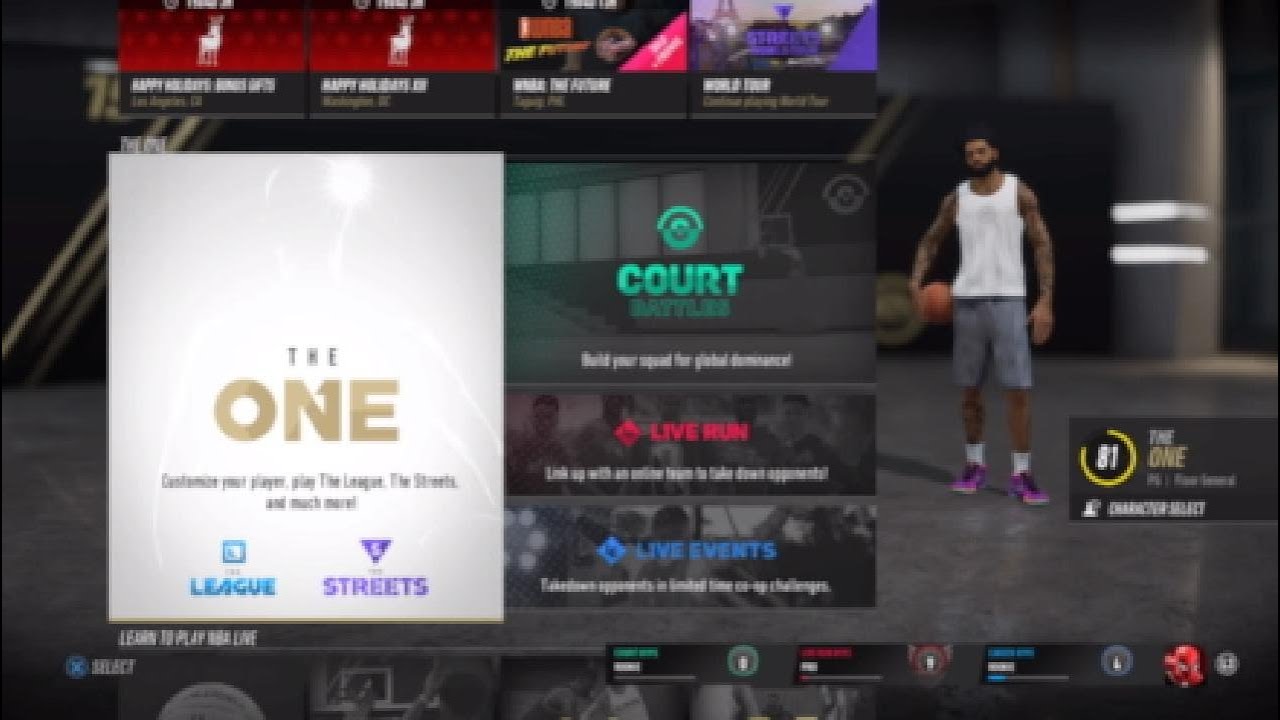The image is a blurry screenshot from a video game, featuring a character select screen. 

In the background, there's a dark grey, reflective cement surface leading to a distant grey wall, adorned with golden stripes angled from the bottom left to the upper right. 

Positioned on the right side of the screen is a basketball player. He is dressed in a white tank top, short grey shorts, white socks that reach halfway up his calves, and pink shoes with black laces. He has a black beard, short black hair, and is holding a basketball with his right hand at his right hip.

In the lower right corner, there is a translucent dark grey pane. This pane contains a black circle on the left with the white number "81" at its center, surrounded by a yellow outline forming a three-quarters enclosed "C" shape from the 12 o'clock to the 9 o'clock positions. To the right of the circle, the player's name appears, but it is too blurry to read. The name is displayed in italicized text, with the first name in white and the last name in gold beneath it. Below the name, in white text, it reads "Character Select," accompanied by a white icon of a person to its left.

On the left side of the screen, there is another pane divided into several sections. The entire left portion is occupied by a very light grey background with a faint outline of a person on it. Adjacent to it are three horizontal rectangles with dark grey backgrounds. The top rectangle has blue text reading "Court Battles," the middle rectangle has red text stating "Live Run," and the bottom rectangle has blue text reading "Live Events." On the far left is a white pane with the text "The One" in gold.